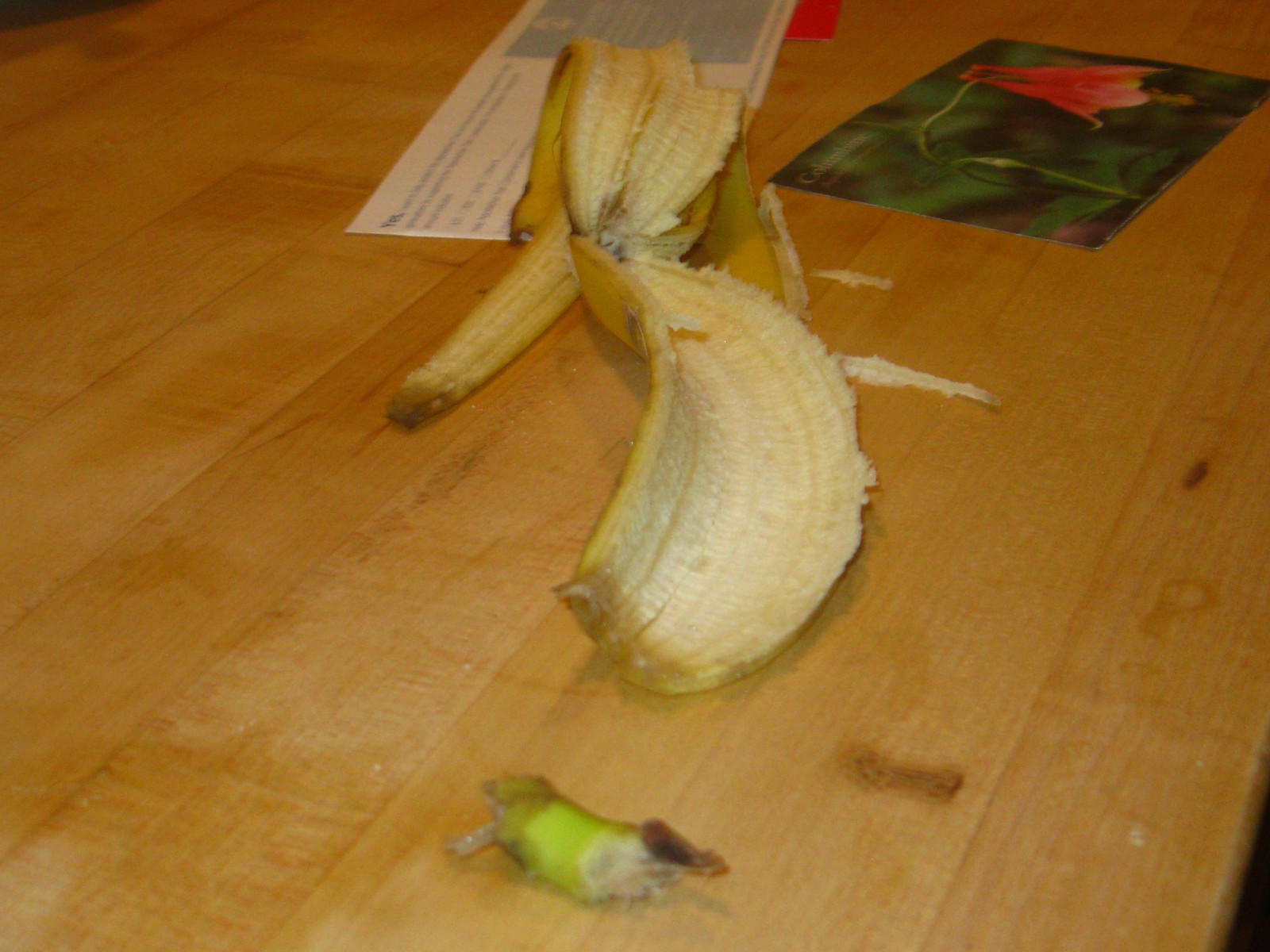This photograph features a light blonde wooden table that dominates the frame, with a few dark spaces in the top left and bottom right corners that hint at the floor or another surface below. The main subject on the table is an empty banana peel, positioned with its inside facing up and slightly folded at the back. The green top stem of the banana, broken off from the peel, lies a few inches below it on the table. In the upper right corner of the image, there appears to be a printed postcard depicting an orchid. The flower has a green stem that angles upward to the right, with a bell-shaped blossom hanging beneath it. Beneath the banana peel is a white card that might be a flyer, possibly from a power company, lying flat on the table. The table's light blonde wood has a yellowish tone, adding warmth to the scene.